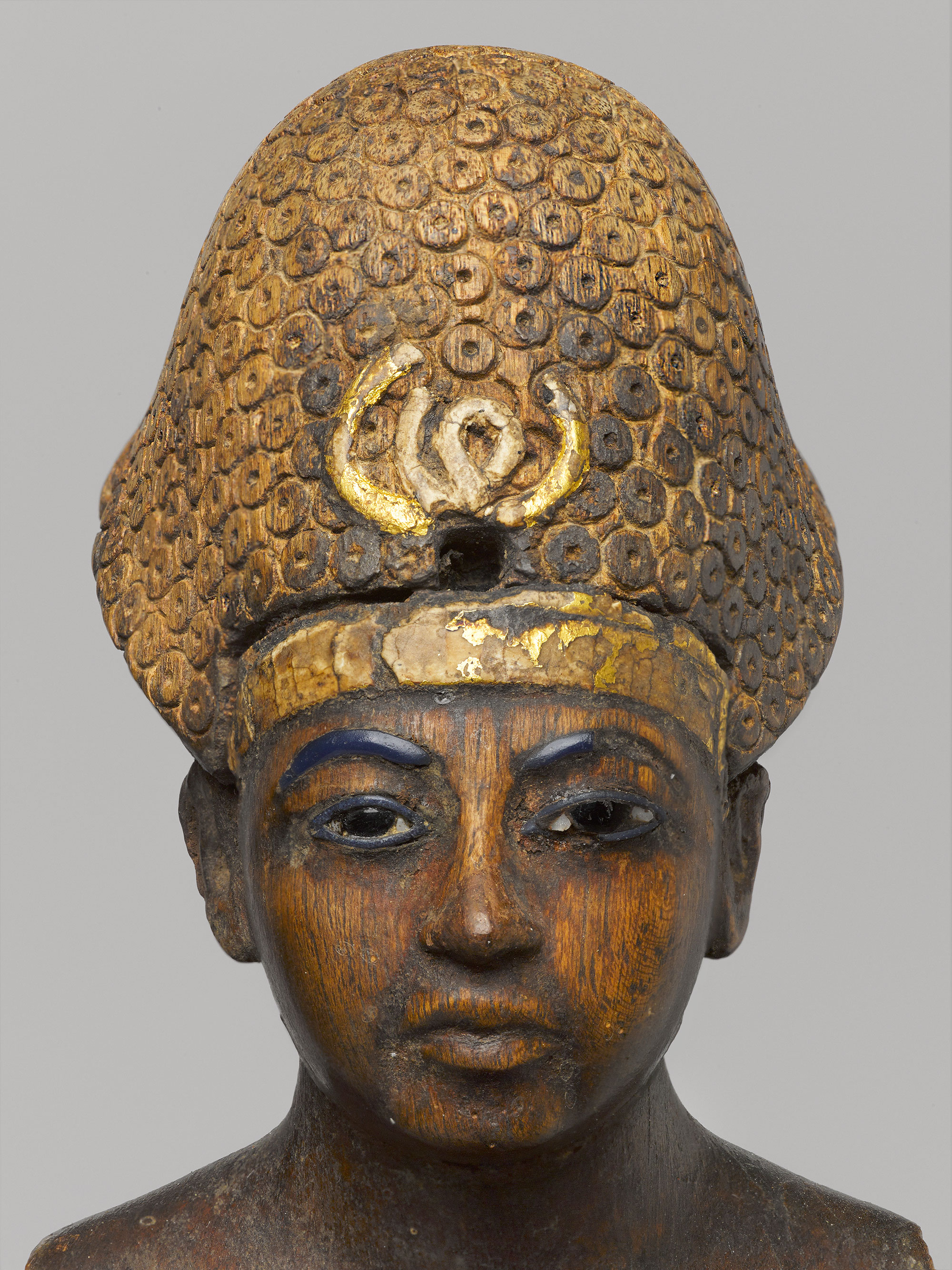This photograph captures a meticulously carved wooden bust, likely representing an ancient Egyptian figure, possibly a pharaoh or an African princess. The statue is predominantly made of dark wood with a rich grain, deepening the lifelike quality of the image. The figure wears a grand, bulbous headdress that flares out at the sides and tapers towards the top, richly adorned with circular patterns reminiscent of carved-out cheerios or washers. This unique texture gives the headdress a striking three-dimensional effect. 

A prominent golden headband encircles the forehead, accentuating a symbolic gold swirl or crest at the front, which might hint at regal affiliations. The headdress appears to have a faded teal shade, with darker shadows enhancing its depth. The face of the statue features jet-black eyebrows and almond-shaped eyes, highlighted by black eyeliner, which imbues the bust with an intense, straight-ahead gaze. The delicate nose, pursed lips, and carved ears further add to the statue's realism, reflecting the sophisticated artistry of ancient times. The bust is finely detailed down to the shoulders, set against a plain gray background, which helps to focus attention on the intricate features and regal adornments of the figure. 

Overall, the statue suggests an artifact of significant historical value, possibly originating from a museum collection, and stands as a testament to the rich cultural and artistic heritage of ancient civilizations.